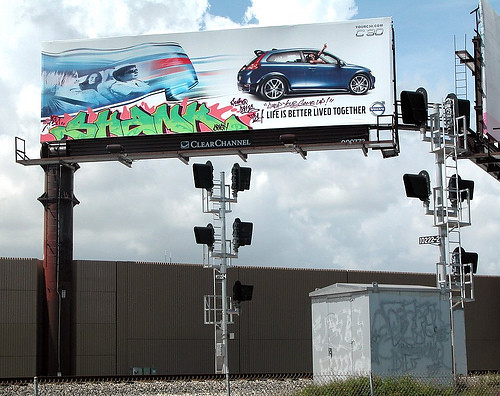The image depicts an industrial area featuring a prominent billboard positioned above a set of railroad tracks. The billboard advertises a Nissan SUV, possibly a model labeled either C30 or C50, depicted in a vibrant blue color and oriented towards the right. The vehicle's tagline reads "Life is better lived together," and suggests an atmosphere of camaraderie and adventure, showing a passenger enthusiastically sticking their hand out, as if to evoke the spirit of a dynamic journey. The left side of the advertisement displays a somewhat abstract, blurry depiction perhaps illustrating an interior view of the car.

The lower third of the billboard is heavily graffitied, with the word "Shank" or "Skank" scrawled in bold green gradient text accompanied by a blobby red-pink and black background, adding to the overall gritty urban aesthetic. The environment surrounding the billboard includes a gray cement shed, railroad traffic lights, and scattered graffiti on various surfaces, emphasizing its industrial setting. Additionally, there is a nearby structure that resembles a storage shed or a transformer box, similarly adorned with tags. A large brick wall and an empty billboard frame loom in the backdrop. The scene is bathed in natural light, suggesting it was taken on a clear day with a blue sky dotted with clouds.